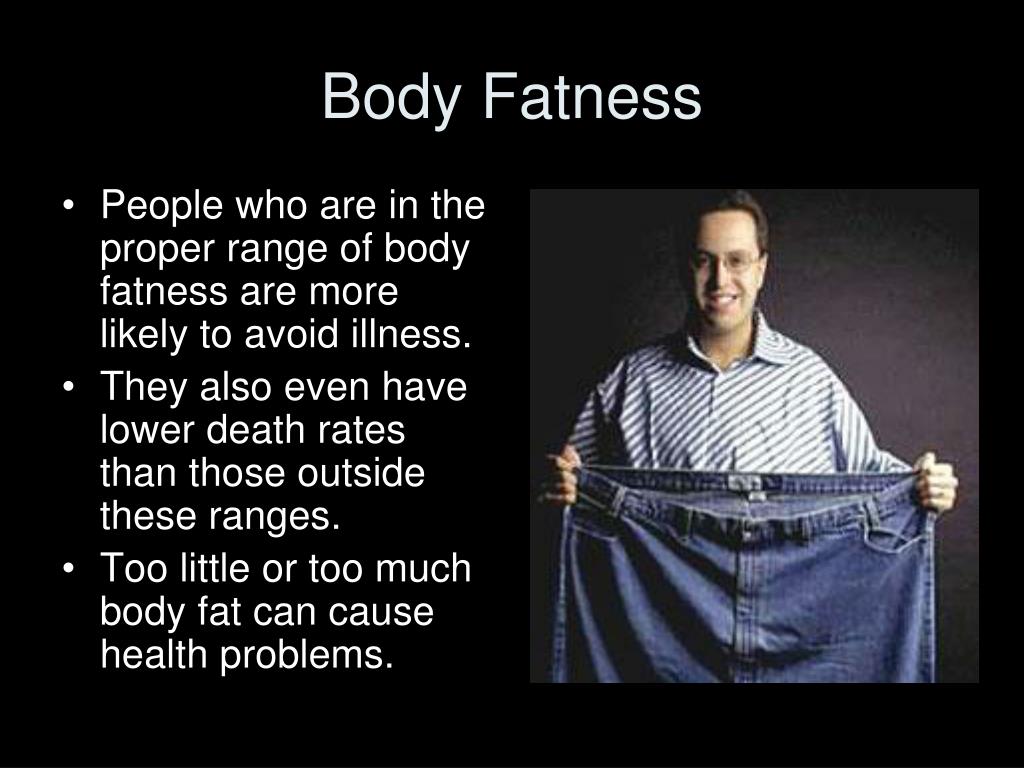The slide appears to be from a PowerPoint presentation, featuring a black background with white writing. The title at the top reads "Body Fatness" in large, white font. On the left side, there are three bullet points in white text: 
1. "People who are in the proper range of body fatness are more likely to avoid illness."
2. "They also have lower death rates than those outside these ranges."
3. "Too little or too much body fat can cause health problems."

On the right side of the slide, there is an image of Jared from Subway, a white man with brown hair and glasses, smiling at the camera. He is wearing a diagonally striped button-up shirt and is holding a very large pair of jeans, presumably from before he lost weight. The background behind Jared is a mix of black and grayish tones.